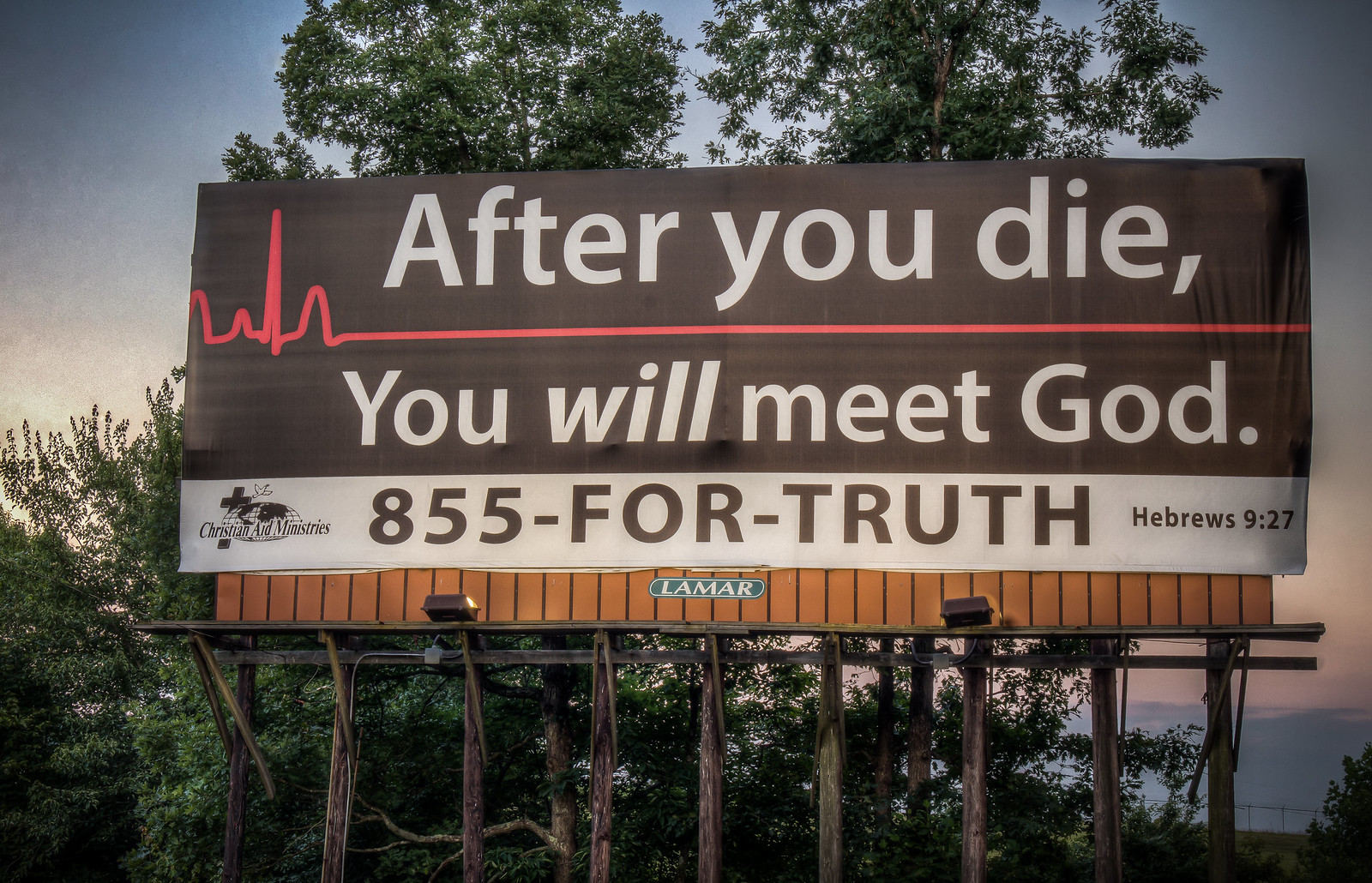A large roadside billboard dominates the photograph, framed by what appears to be the soft light of either sunrise or sunset, casting blue and pink hues across the sky. The hilly landscape in the background, complete with green trees directly behind the billboard, adds to the serene yet somber atmosphere. The billboard itself features an EKG heart monitoring line running down the middle, illustrating the lifeline as it rises and falls, ultimately flatlining. Above the EKG line, a poignant message in white font against a brown background reads, "After you die," while below it, the text solemnly proclaims, "You will meet God." The bottom left corner indicates that this message is brought to you by Christian Aid Ministries, accompanied by a phone number for contact. Additionally, the billboard references a Bible passage from Hebrews 9:27, further emphasizing its religious context.